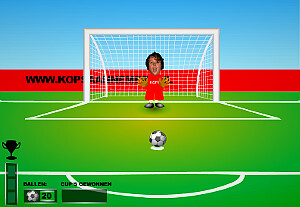The screenshot captures a vibrant moment from a soccer video game. In the image, a player wearing a red jersey and red shorts attempts to shield his face with his hands as he positions himself near the soccer goal. His curly hair partially obscures his face, emphasizing the dynamic movement of the scene. The green turf, marked with white lines, clearly indicates a soccer field. A crisp white net stands behind the player, adding to the realism of the virtual match. 

A red banner in the background suggests the presence of in-game advertisements or sponsorship placements, typical in sports venues. A soccer ball hovering on the field with a white circle underneath it confirms its digital nature. At the bottom of the image, a trophy symbol accompanied by the text "Ball Ball 20" can be seen, indicating a potential game achievement or progress tracker involving 20 soccer balls. Additionally, there's a slightly ambiguous section displaying "Cups Gin one," which might be a garbled display or an incomplete text. A long black rectangle, possibly a user interface element, stretches beneath this information. The sky above the stadium is a clear blue, adding a touch of realism and cheerfulness to the overall scene.